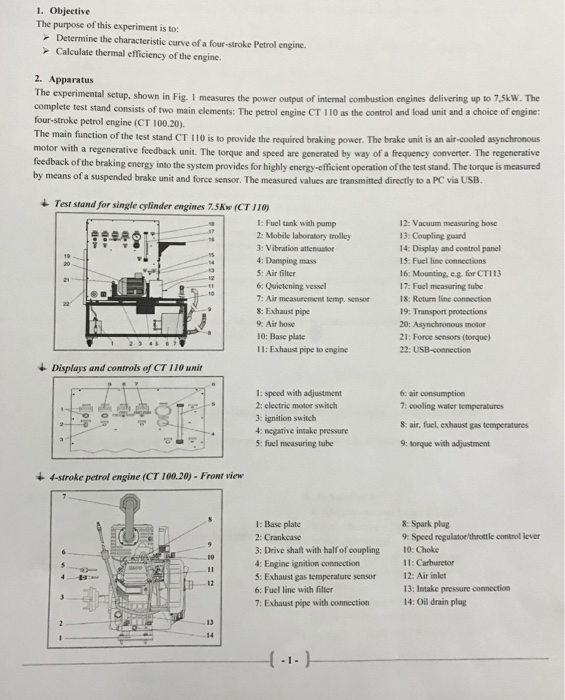The image appears to be a black-and-white photograph of a scientific instruction manual or student paper. At the top of the page, there is a section titled "Objective," stating that the purpose of the experiment is to determine the characteristic curve of a four-stroke petrol engine and calculate its thermal efficiency. Below this, there is an "Apparatus" section detailing the components of the experimental setup. This setup includes a petrol engine CT 110, which serves as a control and load unit for four-stroke petrol engines like the CT 100.20, capable of delivering up to 7.5 kW of power. The apparatus description also highlights a regenerative braking air-cooled asynchronous motor, with values transmitted via a PCVUSB display unit.

Beneath the descriptive text, the page features several black-and-white illustrative diagrams with numbered parts, each labeled and listed to the right of the images. Among these diagrams, one depicts the test stand and labels components such as the fuel tank with pump, mobile laboratory trolley, and air filter. Another diagram focuses on specific engine parts like the crankcase, engine ignition connection, and exhaust gas temperature sensor. The diagrams are enclosed in black-and-white squares and meticulously detail over 22 parts in one and nine in another, while the four-stroke petrol engine diagram features 14 different labels.